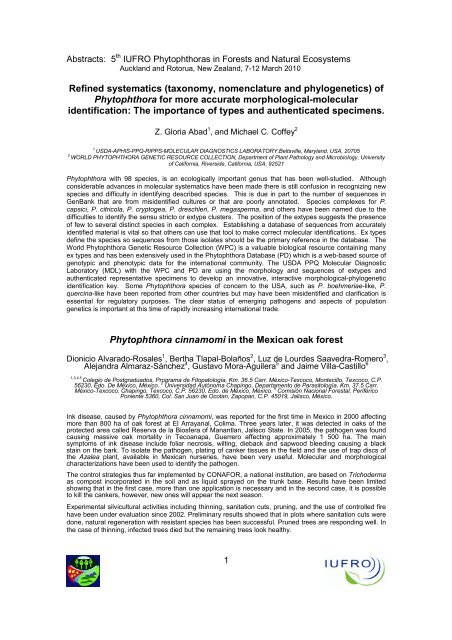The image displayed is a computer screen featuring a scientific article on a white background with finely printed black text. Some sections are emphasized with bold type. The text includes terms such as "abstracts," "iUFO," "FATA," "forest and natural ecosystems," "Auckland," and "New Zealand." In bold, it highlights critical topics like "refined systematics, taxonomy, nomenclature, and phylogenetics of Phytophthora for more accurate morphological and molecular identification, the importance of types, and authentic specimens." Towards the bottom right of the article, there's a blue square containing green images and the word "iUFO," accompanied by a swooping green and blue logo. The article appears to discuss various aspects of ecological systems.